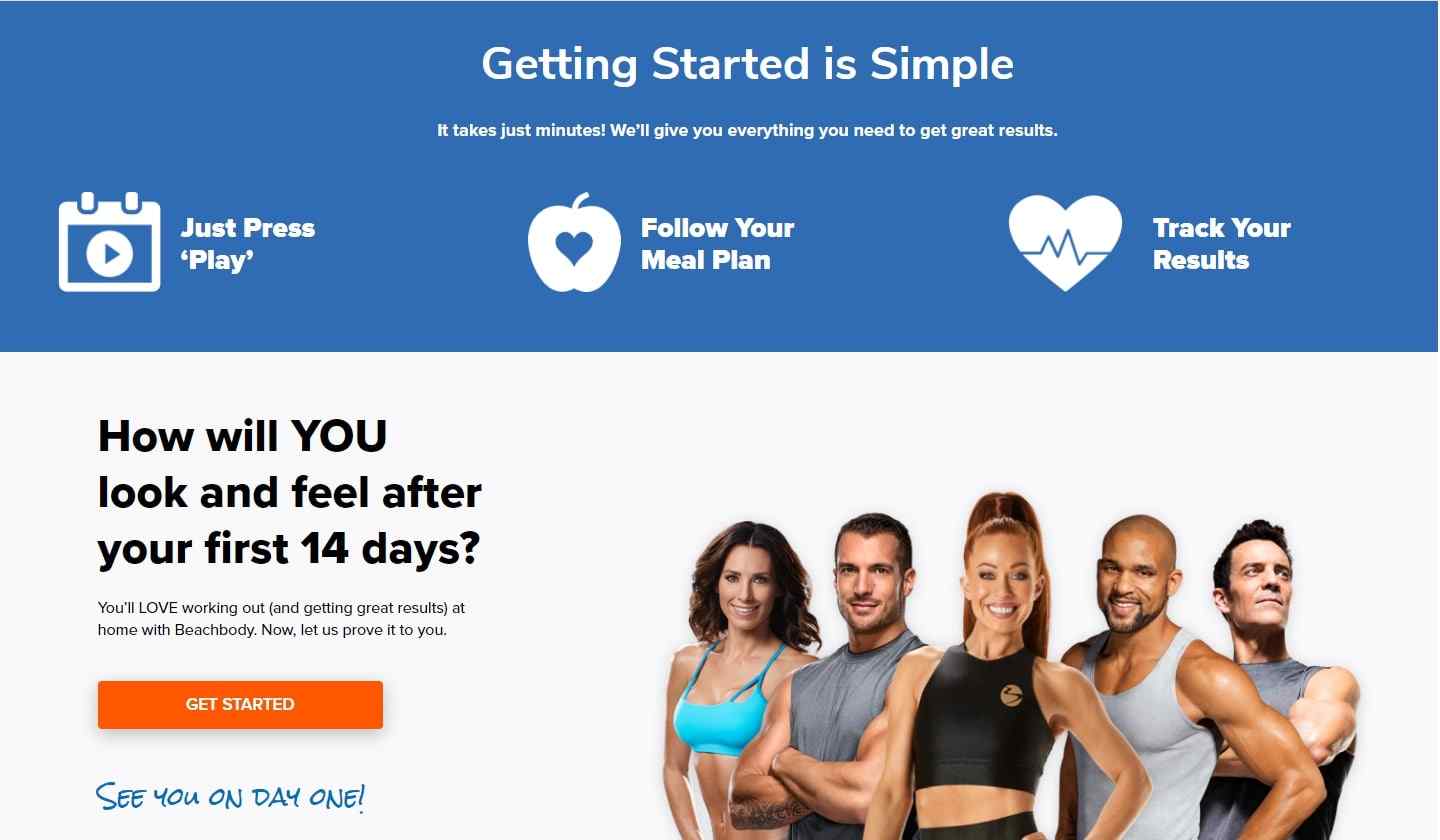The image depicts a promotional advertisement for the Beachbody fitness app. At the top of the image, there is a blue rectangular box, approximately three to four inches in width. The box contains the text: "Getting started is simple. It takes just minutes. We'll give you everything you need to get great results." In the bottom-left corner of this blue box, there is a "Just Press Play" button depicted inside a calendar icon.

In the center of the image, there is an apple graphic with a heart symbol inside, accompanied by the text "Follow your meal plan." To the right of this, there is a heart icon with a 2kg graph, along with the text "Track your results" in white.

The bottom section of the image features a white box. On the left side, it asks, "How will you look and feel after your first 14 days?" followed by the statement, "You'll love working out and getting great results at home with Beachbody. Now let us prove it to you." Below this text, there is an orange "Get Started" button with the text "See you on day one."

To the right side of the bottom section, there are images of happy and fit individuals posing and smiling, showcasing the positive outcomes and community aspect of using the Beachbody app.